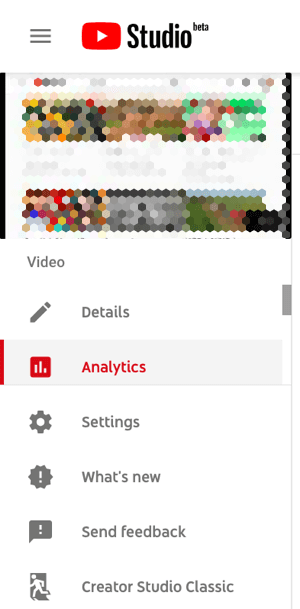A vertically-oriented screenshot appears to be taken from a smartphone screen, though it could also be a heavily cropped section of a PC screen. At the top of the screenshot, there’s the distinctive YouTube icon—a red rounded rectangle with a white play triangle inside. Next to the icon, the text "Studio" is visible, with a superscript "Beta" indicating this is an early access version of the platform. To the left of the YouTube icon is the ubiquitous hamburger menu icon, signifying additional options or navigation.

Below this header, there is an intriguing array of colored hexagons. These hexagons likely represent some form of data visualization, possibly illustrating the color balance over time in the analyzed video, although the exact nature of the diagram is unclear.

Further down, a menu bar showcases several tabs: "Videos," "Details," "Analytics," "Settings," "What's New," "Feedback," and "Creator Studio Classic." Each tab offers different functionalities and insights for video creators. The overall layout and components suggest a user interface designed for video management and analysis.